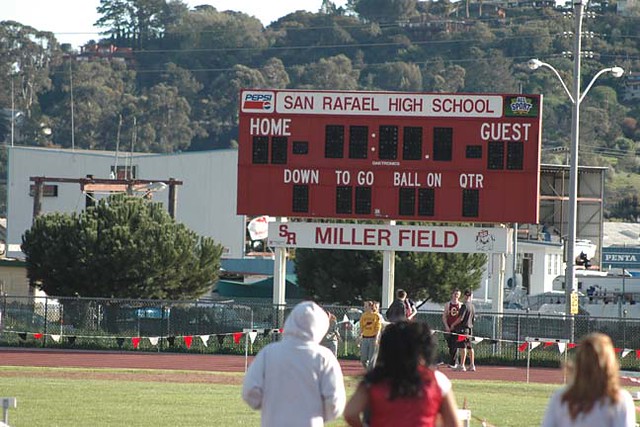This photograph captures an outdoor scene on the school playing field at San Rafael High School. The image is framed with a backdrop of trees and small construction-like buildings far in the distance, as well as a street lamp and a gate enclosing the field, with bushes behind it. The prominent feature is the large, dark red scoreboard, which displays a white banner with red text reading "San Rafael High School" at the top. The scoreboard includes sections for "Home" and "Guest" scores, as well as placeholders for the down, yard, quarter, and additional game information. The top left corner of the scoreboard is marked by a small Pepsi logo. Below the scoreboard, a rectangular white sign with red text indicates "S.R. Miller Field," accompanied by a cartoon dog illustration. The scoreboard structure is supported by a post anchored into the ground.

In the foreground, three people stand with their backs to the camera: one wearing a white jacket with the hood pulled up, an African-American woman in a red shirt, and another woman with blondish-brown hair in a white shirt. All eyes appear to be focused on the field. Nearby, four others are seen conversing and standing around the scoreboard. Red, black, and white triangular plastic decorations are strung around the scoreboard area, enhancing the scene.